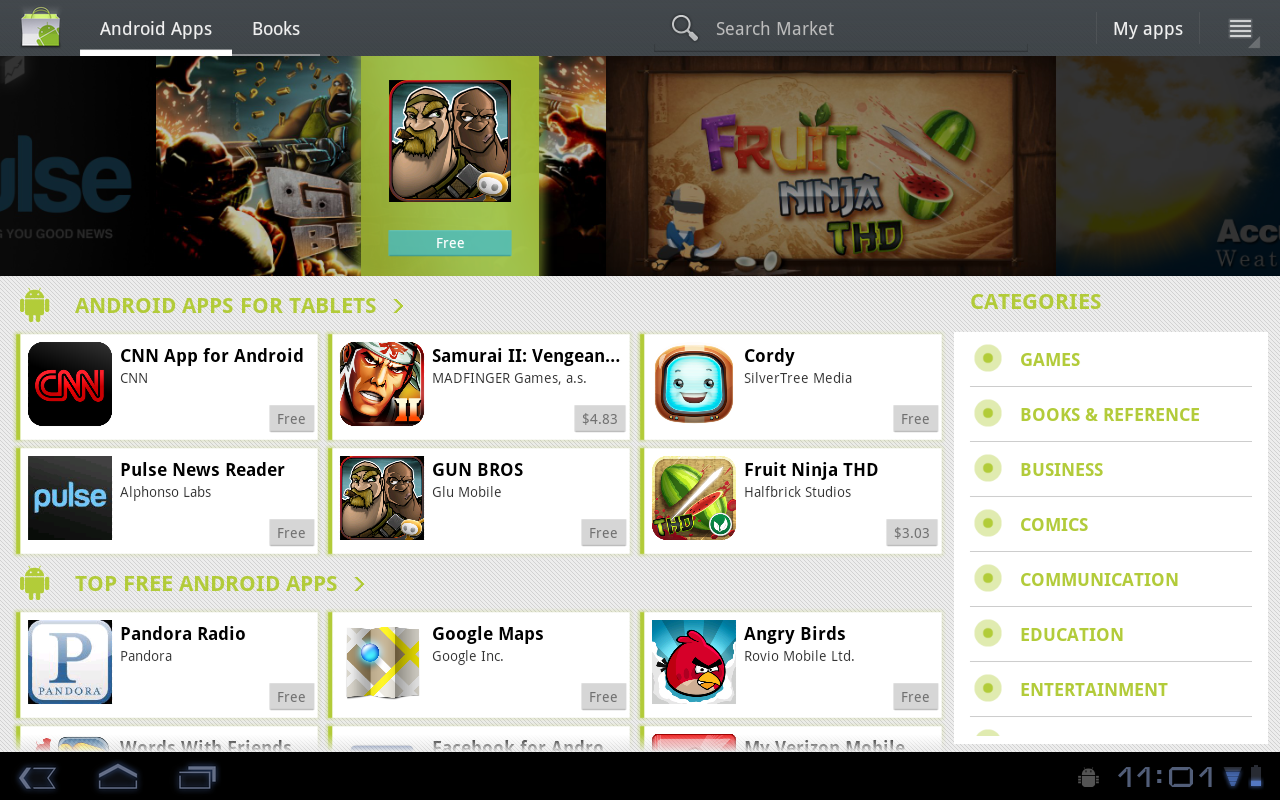This image is a screenshot depicting the layout of the Android tablet app marketplace. On the left side, a navigational tab is visible with "Android apps" currently selected and highlighted with an underline in white. Next to this tab is a "Books" tab indicating other categories available in the marketplace.

The header section features a showcase of various games, with the first game appearing to be a boxing game and the second being "Fruit Ninja HD." Directly below this header, there is a prominent green Android icon accompanied by the text "Android apps for tablets" also in green. 

In the main content area, there are six featured applications listed. These include:
1. CNN app
2. Pulse app
3. Samurai 2
4. Gun Bros
5. Cordy
6. Fruit Ninja THD

Following this section, there is an additional category titled "Top Three Android Apps," marked by a green header with another Android icon. Listed under this category are:
1. Pandora Radio
2. Google Maps
3. Angry Birds

On the far right side of the screen, a "Categories" list is displayed in green text. The categories include:
1. Games
2. Books and References
3. Business
4. Commerce
5. Communication
6. Education
7. Entertainment